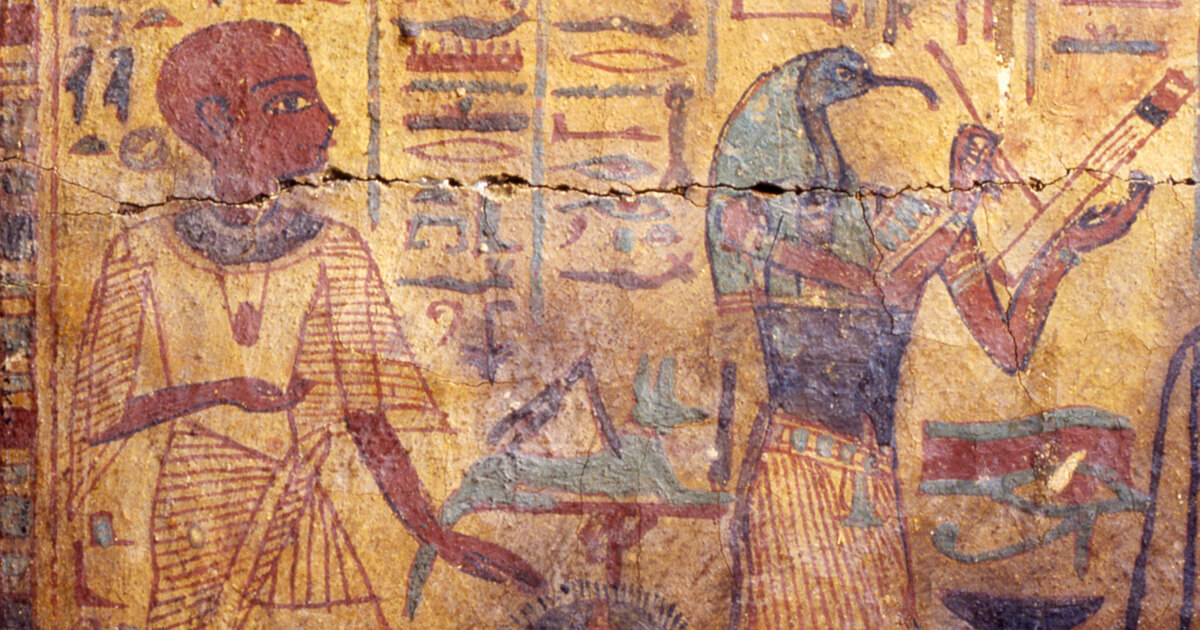This close-up photograph captures an aged and detailed mural, likely part of an Egyptian excavation project, possibly located in North Africa. The painting, set against a yellow-hued stone background, depicts two figures rendered in an ancient hieroglyphic style, complete with surrounding hieroglyphs. A large but unobtrusive crack runs through the middle of the mural, adding to its timeworn character.

On the left, a human figure with dark brown skin is adorned in a white robe and an orange pendant necklace. This individual is presented with a head in profile, gazing to the right while their body faces forward. One arm is bent across their midriff, and the other rests at their side.

Next to them is a distinguished figure with the head of an ibis, featuring a distinct black curved beak. This entity, depicted with black skin, wears a traditional green Egyptian headdress that drapes down the back. Clad in a sleeveless black shirt and a white skirt, the ibis-headed figure appears to be writing on a papyrus scroll with a stylus. Additional elements enrich the mural, including a blue headdress, an outline of a blue eye, and a blue cat sitting on a table, enhancing the intricacy and cultural significance of the scene.